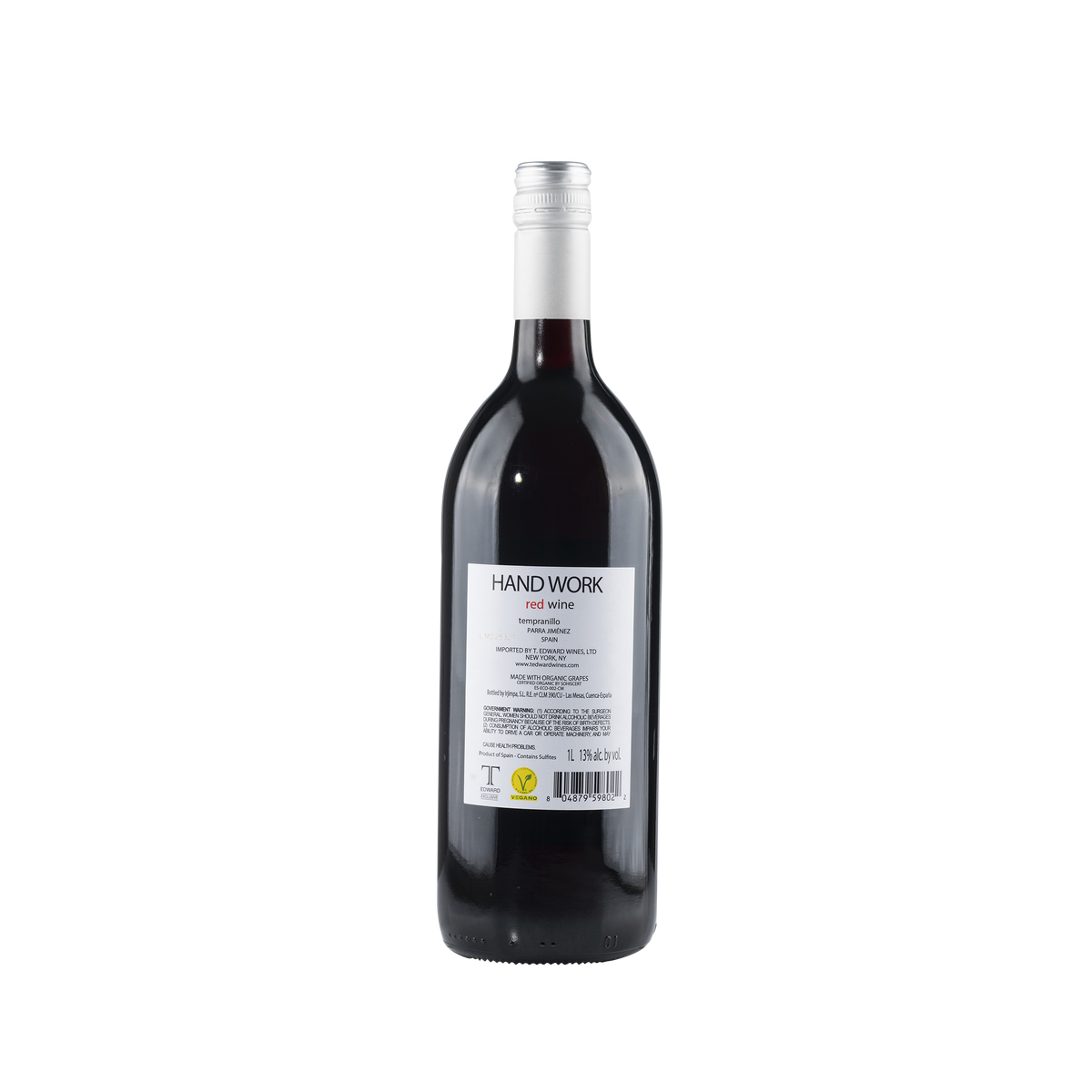The image depicts a single bottle of red wine against a pristine white background. The wine bottle features a label prominently displaying the name "Handwork, Red Wine, Tempranillo." The label notes the alcohol content as 13% by volume and indicates that the bottle contains 1 liter of wine. Additional text on the label mentions "New York, New York," alongside a government warning. A barcode is visible on the bottom right of the label. The bottle itself has a sleek design with a silver cap and a silver neck, contrasting against the dark red wine inside the glass bottle.